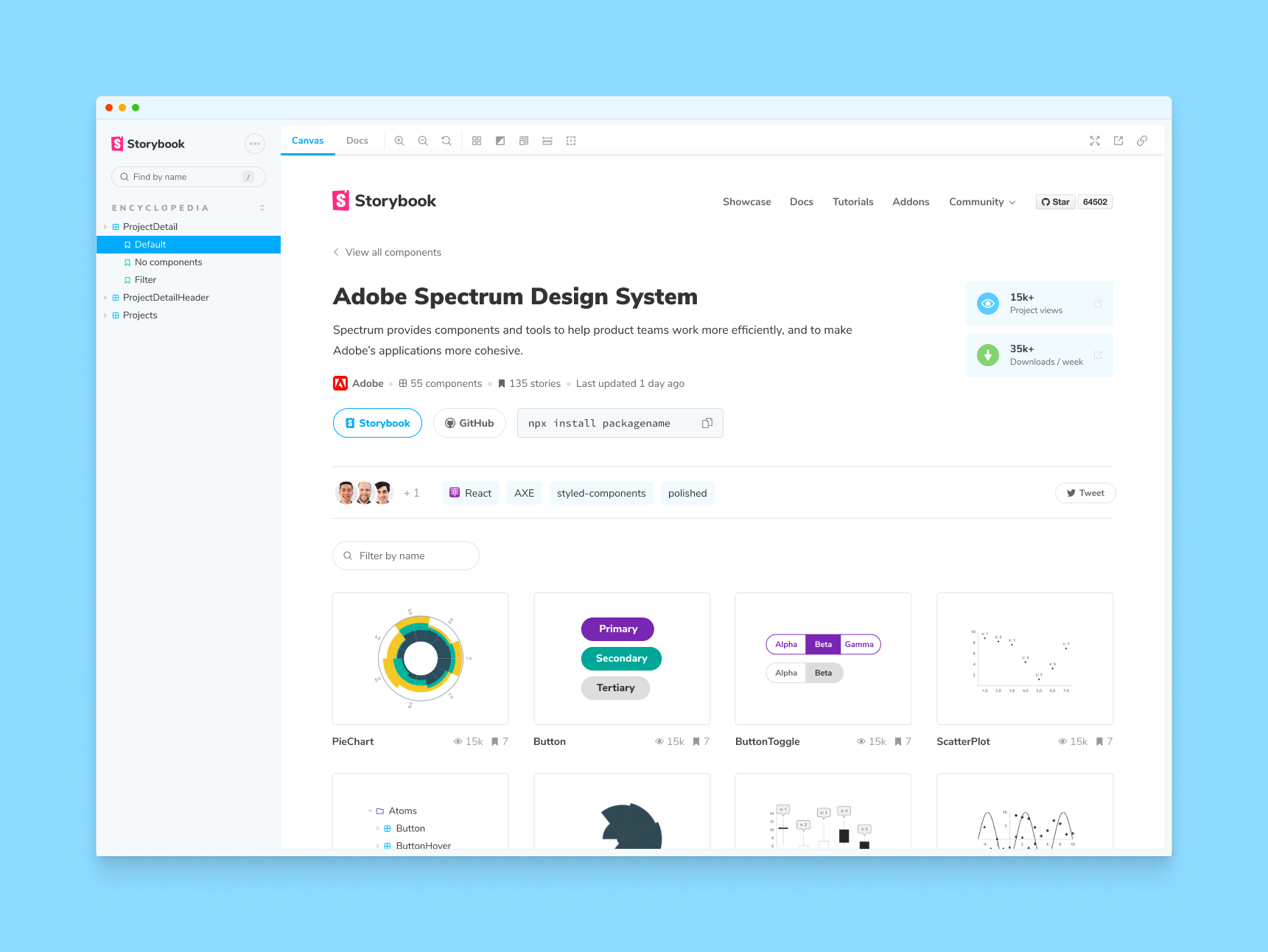This screenshot captures a vibrant, light turquoise user interface from an unidentified website. At the heart of the image is a prominent white window. To the left, there's a vertical navigation menu listing options: Storybook, Find by Name, Encyclopedia, Project Detail, Default, No Components, Filter, Project Detail Header, Projects. 

On the right side of the window, several headings and statistics are displayed, creating a dense, information-rich sidebar. It includes "Storybook," "Showcase," "Docs," "Tutorials," "Add-ons," and "Community." The section also proudly displays a 'Star' icon followed by the number '64,502'. Additional options like "View All Components" and "Adobe Spectrum Design System" are present as well, with a descriptive note: "Spectrum provides components and tools to help product teams work more efficiently and to make Adobe's applications more cohesive."

Further details outline Adobe's resources: "55 components, 135 stories, last updated one day ago." Links to "Storybook," "GitHub," and an "NPX Install Package Name" for React are also indicated. Metrics showcasing user engagement feature the entries "AXE," "Styled Components," "Polished," "15,000+ project views," and "35,000+ downloads a week." At the bottom, abbreviated elements such as "Tweet," "Filter by Name," "Pie Chart," "Button," "Button Toggle," and "Scatter Plot" are partially visible, hinting at various functionalities and features that extend beyond the captured frame.